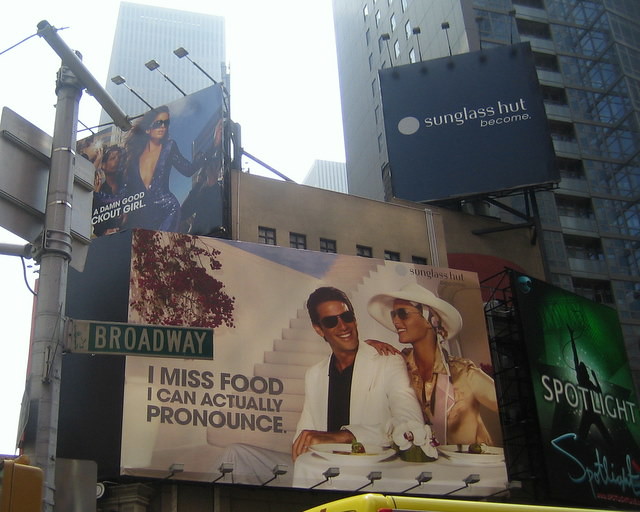The image depicts a series of four vibrant billboards in an urban area, characterized by towering skyscrapers in the background. 

1. The top left billboard displays an advertisement with the slogan "A damn good something", featuring several women adorned in elegant dresses, one wearing glasses. The scene is bustling with people seemingly taking photos, set against a backdrop of a clear blue sky.

2. Below this, the bottom left billboard showcases a man in a white suit and black shirt, paired with sunglasses. A woman stands beside him with her hand on his shoulder, wearing a white hat and a yellow shirt. They appear to be enjoying a meal, as indicated by the white bowls and table, with a plant and stairs in the background. The caption reads "I miss food I can actually pronounce".

3. The top right billboard presents a sleek, black background with the words "Sunglass Hut" prominently displayed.

4. Adjacent to it, the bottom right billboard features a dramatic image of a silhouetted man against a spotlight, enveloped by a white light and set against a green background. The overall composition captures the essence of urban sophistication and dynamic advertising.

To the left of these billboards, a street pole bears a sign reading "Broadway", firmly situating the scene in a bustling metropolitan setting.